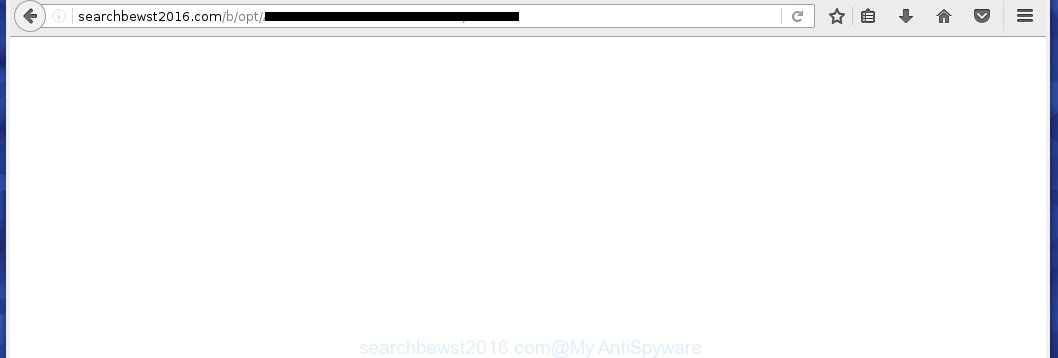This image captures a screenshot of a web browser displaying the URL "bewest2016.com/be/opt/redacted" on a blank white page. At the top, a gray navigation bar features several buttons: a refresh button, a favorites button, a paste button, a download button, a home button, and a menu represented by three lines. Additionally, a back button is located to the left of the web address. The bottom of the page displays the text "search bewest2016.com at my antispyware." Vertical blue bars frame the left and right sides of the screen, providing a visual boundary for the otherwise unoccupied white space.